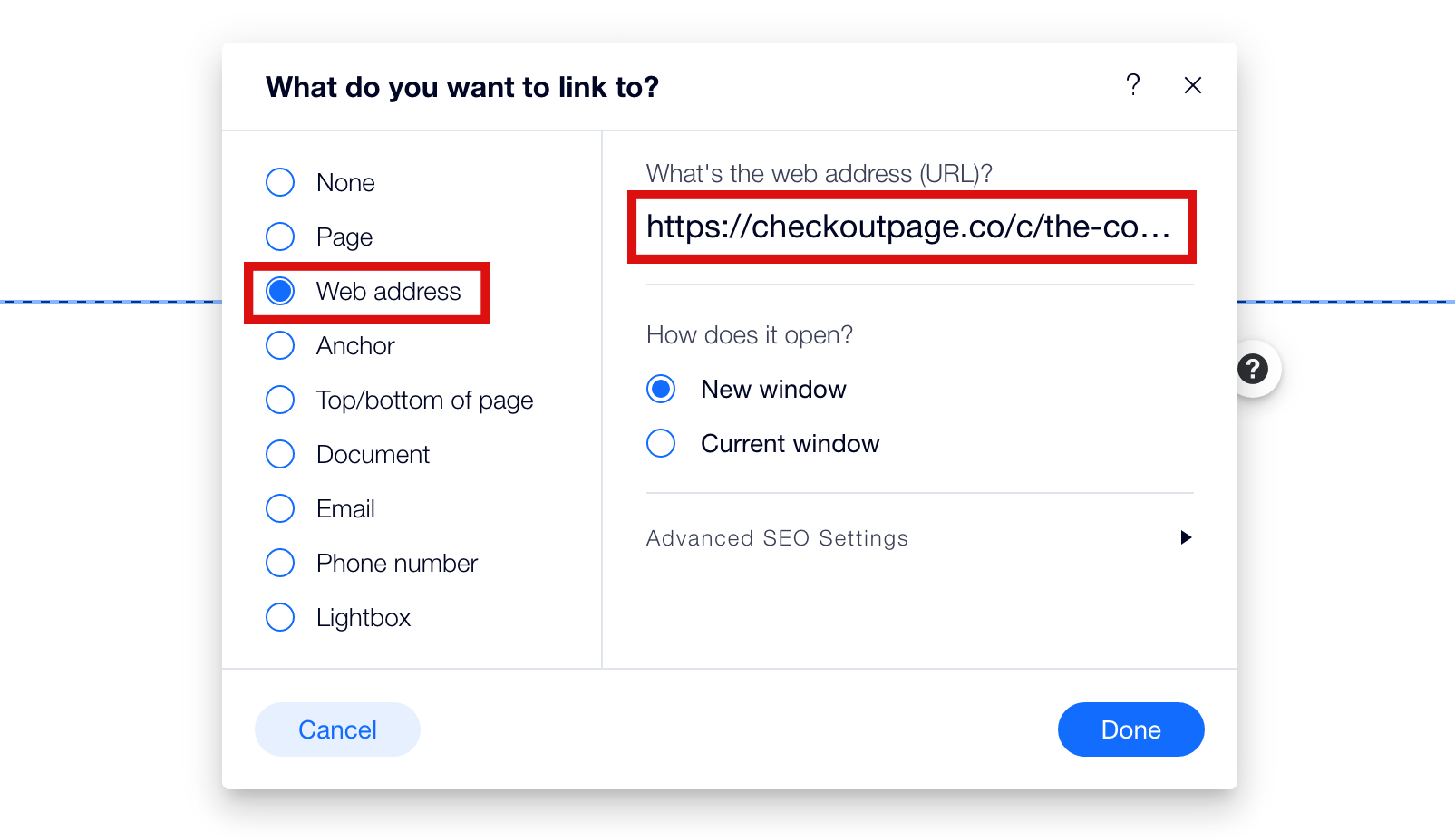A pop-up window has opened, obscuring the view of the page behind it. The underlying page is marked by a blue dotted line with an element partially visible in the middle, appearing as a small white disc encircled by a gray ring, containing a question mark.

The pop-up, titled "What do you want to link to?" features a top bar with an exit option. On the left side of the pop-up, a vertical column lists selectable options: "None," "Page," "Web address" (currently selected), "Anchor," "Top of page," "Bottom of page," "Document," "Email," "Phone number," and "Lightbox." 

To the right, occupying a larger section of the window, is the input field for the web address or URL, labeled "https." Below this, under the label "How does it open?" are two radio buttons for selecting either "New window" or "Current window," with "New window" currently selected. 

Further down, beneath a blue line, is an expandable section labeled "Advanced SEO settings" with an arrow icon for more details, currently unexpanded. At the bottom of the pop-up are two buttons: a "Cancel" button on the left and a "Done" button in blue on the right.